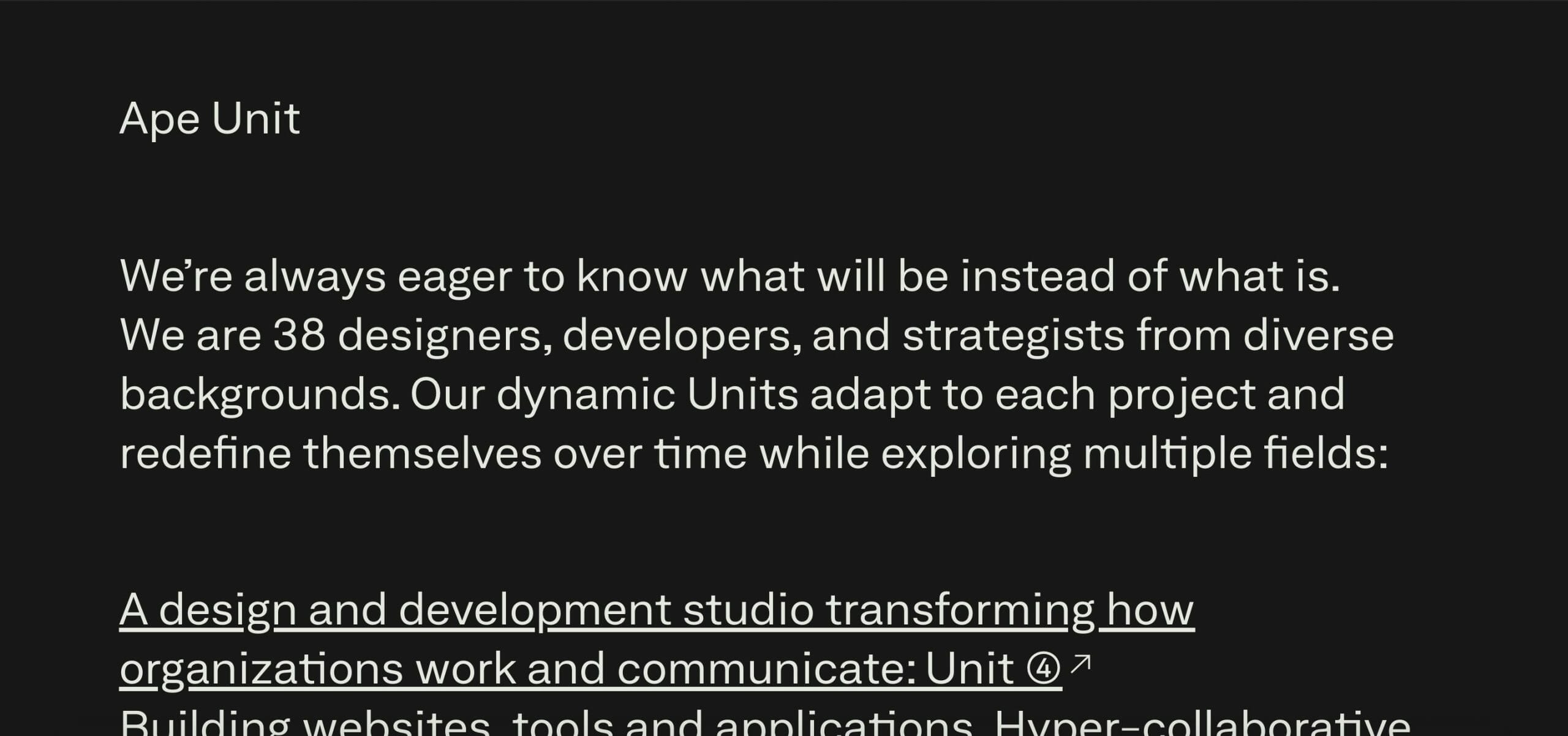The image features a black background with white text. At the top, it prominently displays the words "APE Unit" in white. Below this, a paragraph reads: 

"We're always eager to know what will be instead of what is. We are 38 designers, developers, and strategists from diverse backgrounds. Our dynamic units adapt to each project and redefine themselves over time while exploring multiple fields."

This paragraph is underlined and followed by:

"A design and development studio transforming how organizations work and communicate."

Next, there is an illustrated circle containing the number "4" and an arrow pointing upwards toward the word "how". Underneath this, a truncated sentence is partially visible, with only the tops of the words readable. It appears to say:

"Building websites, tools, and applications. Hyper-collaborative."

However, the bottom part of the text is cut off and unreadable.

The overall presentation lacks specific details about the company, such as its name, location, or contact information. The design conveys a sense of mystery and emphasizes the team's adaptability and collaborative spirit.